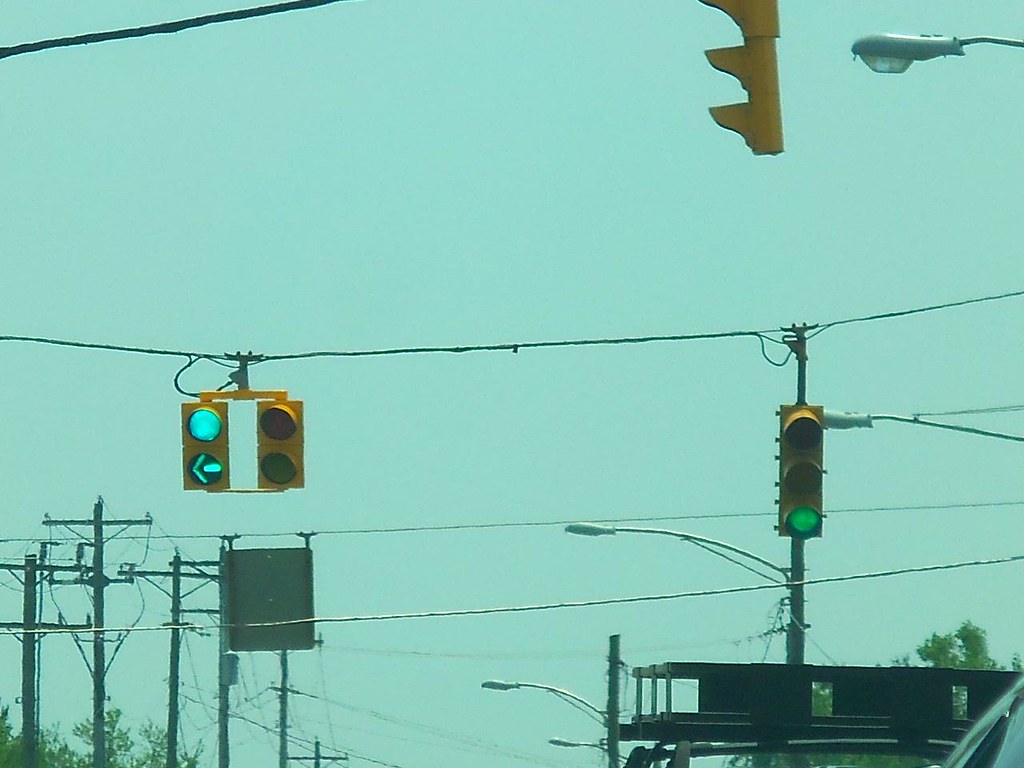In this blurred photograph, taken through a car window, a teal-blue, possibly stormy or sunset sky forms the backdrop, featuring a mix of clouds. The scene is dominated by a network of long utility and electrical wires stretching horizontally across the image. Several telephone poles support these wires, with some sections adorned with streetlights and traffic signals. Prominently, a vertically-hanging traffic light displays a green signal at the bottom. Additionally, two shorter traffic units are visible, each containing two lights with green arrows pointing left at the bottom. The top of a vehicle, potentially a train or a car, is noticeable in the lower right corner, possibly carrying a black ladder on its roof. Silver streetlights are scattered in the distance, adding to the complexity of the scene. The overall image suffers from poor quality, with elements appearing blurry and off-center, emphasizing a somewhat chaotic urban or industrial setting.